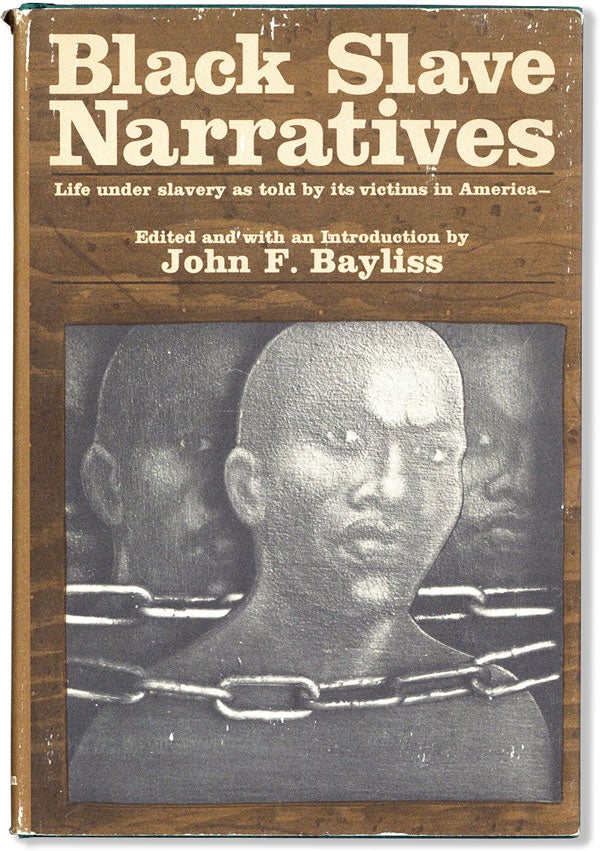The image shows the cover of a book titled "Black Slave Narratives: Life Under Slavery as Told by its Victims in America," edited with an introduction by John F. Bayliss. The title and accompanying text are rendered in a cream-colored font. The book jacket features a brown wood grain design that mimics the appearance of polished wood. Centrally positioned on the cover is a monochromatic (black and white) drawing of a distressed African-American man. He is bald, displaying prominently wide-set eyes, a broad nose, and full lips. The man is depicted without clothing and has two large, loosely hanging chains around his neck, giving him a pensive and concerned demeanor as he makes direct eye contact with the viewer. In the shadowed background, the faint, detailed faces of two other African-American individuals can be seen, also appearing to look in the same direction as the central figure.